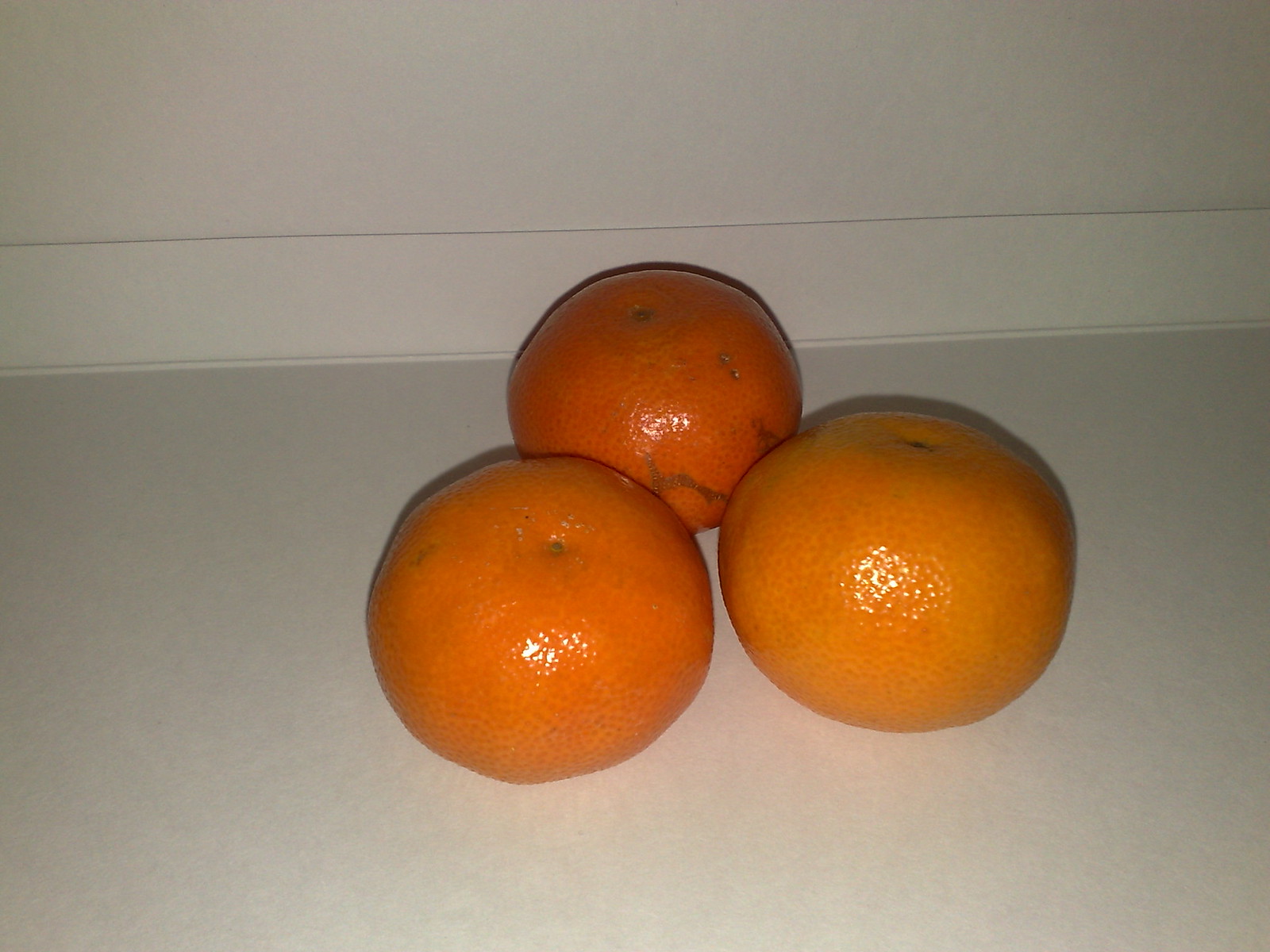This image depicts three fruits that are likely tangerines due to their smaller size and thinner, peelable skin. They are arranged in a triangle formation, with two at the base and one at the apex near the back. The tangerines are positioned on a shiny, creamish-gray countertop, which reflects the warm orange color of the fruits. Behind them is an off-white wall featuring a straight horizontal line, likely a kickboard, about four to five inches from the bottom. The lighting creates a glowing reflection on the tangerines' skin, highlighting their textures and imperfections. The tangerine at the apex has noticeable skin injuries extending towards the bottom, whereas the one on the right appears fresh and unblemished. The bottom left tangerine also has a small scratch on its upper left side. The photograph's bright light source accentuates these details, providing a vivid and detailed presentation of the scene.